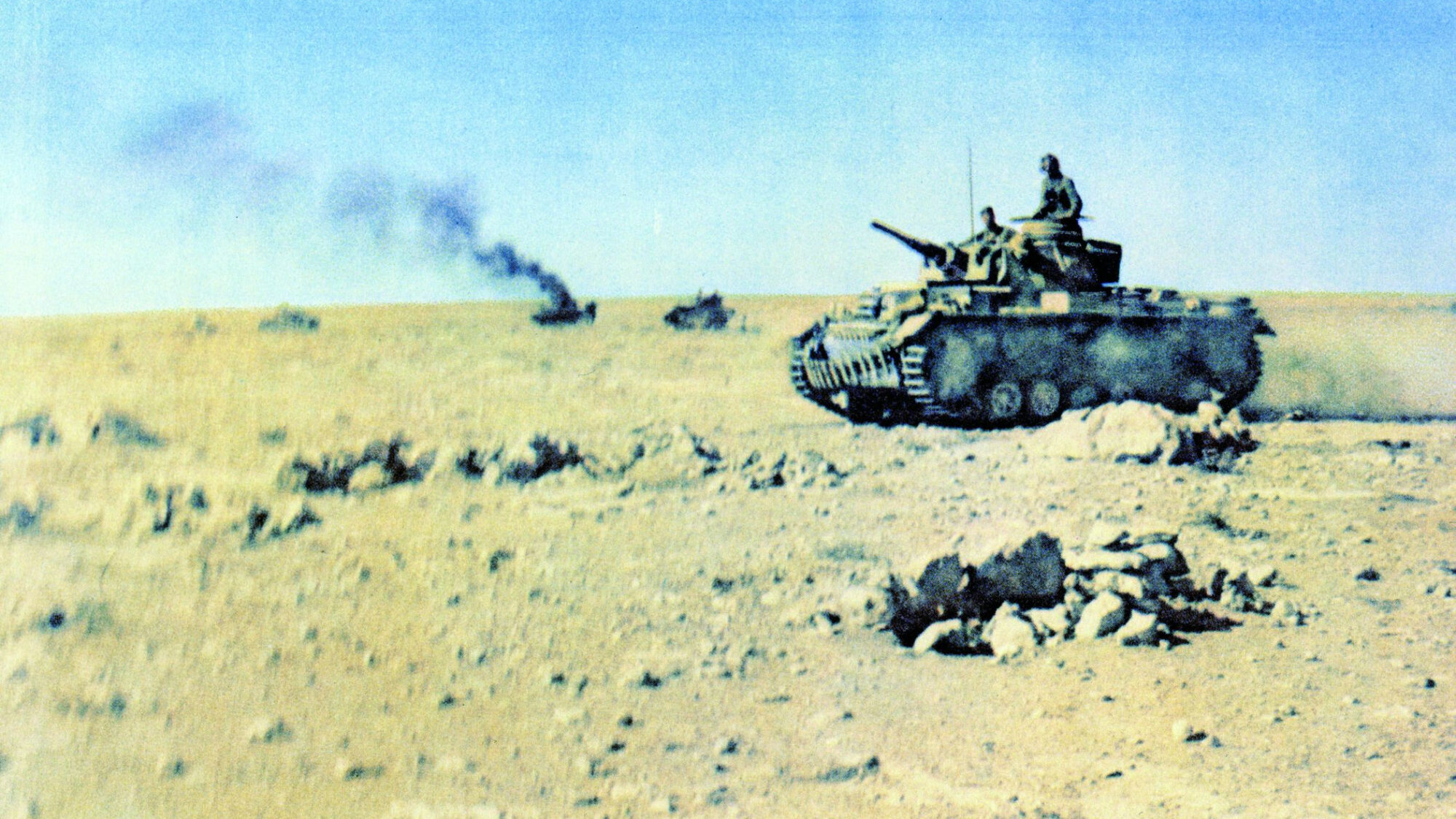The image, a faded and slightly blurry outdoor photograph that appears to be quite old, depicts a desolate battlefield scene. In the foreground, a green military tank moves across a barren, white dirt landscape, which is scattered and piled with white stones, devoid of any vegetation. Two soldiers are visible on the tank; one is manning the cannon on the top, while the other peers out from the open hatch. The background features additional tanks, with one spewing black smoke into the sky, indicating possible damage or destruction. The overall environment resembles a rocky desert, with a few clusters of small stones and a clear, albeit faded, blue sky overhead. The photograph exudes a vintage quality that suggests it could either be a picture taken with an old, low-quality camera or a painting capturing a historical event.